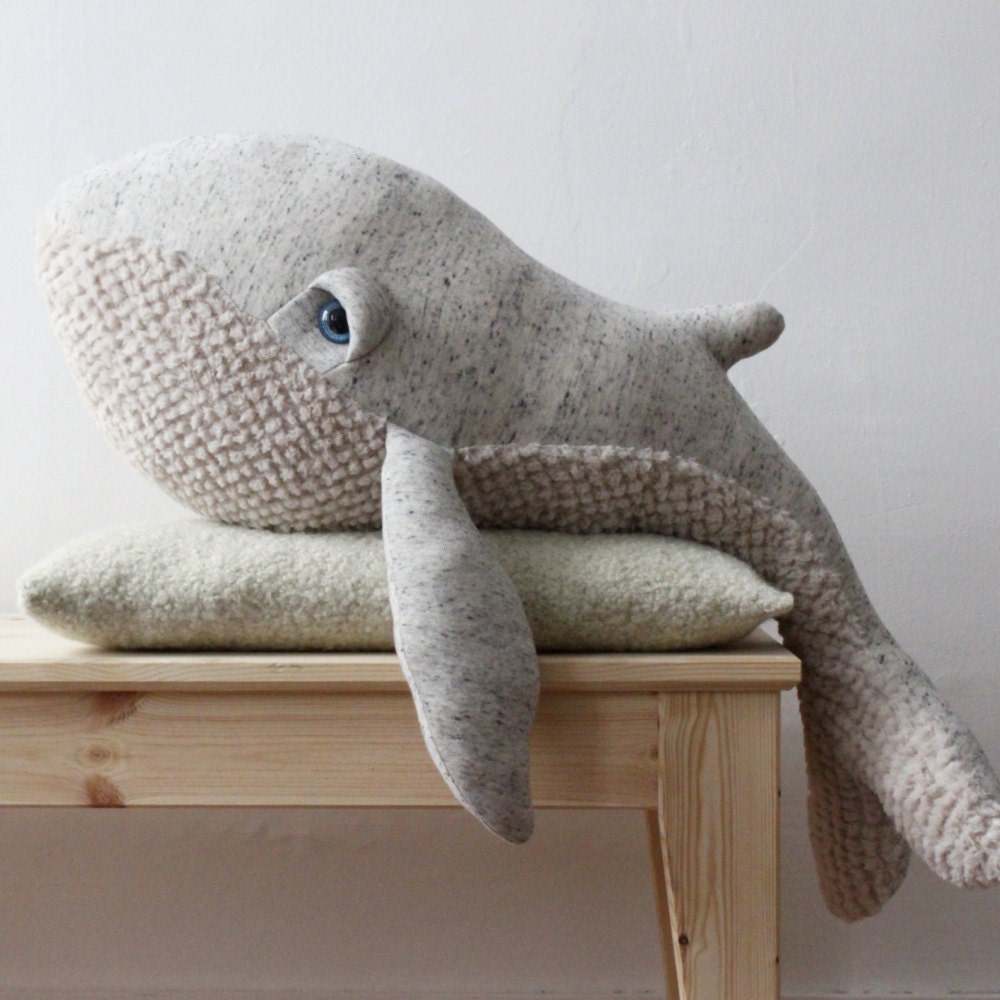The image showcases a charming, gray stuffed whale positioned on the edge of a wooden table, which is light oak or pale pine in color. The whale, likely a high-end toy or handmade, features large blue plastic eyes and has a quilted, woven fabric covering its underside, contrasting with the smooth fabric on its top. Notably, the whale has a peculiar horn protruding where its tail meets its body, adding a unique touch to its design. It rests on a fuzzy-textured pillow, gray or white in hue, that sits on the table up against a light gray or white wall. One of the whale's flippers is seen hanging off the side of the pillow, facing to the left, creating an overall adorable and neutral-toned composition.